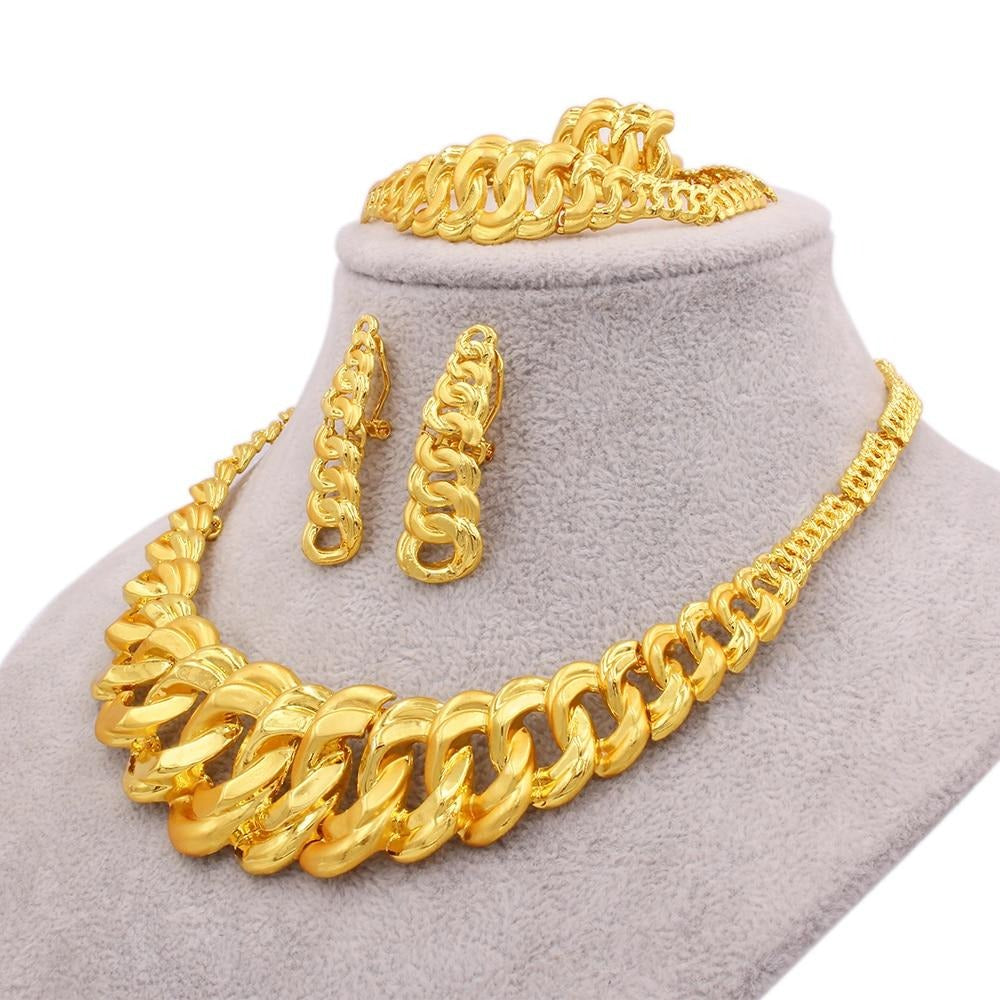This detailed marketing-style photograph features a headless jewelry display mannequin, primarily showcasing an intricate set of gold accessories. The mannequin, which is light cream or gray in color and has a fuzzy texture, is positioned against a starkly white background, making the gold jewelry vividly stand out. The primary focus is a heavy, elaborately designed gold necklace draped around the neck area. The necklace features smaller loops towards the back that gradate into larger, elaborately entwined circles towards the front. Just above this necklace, placed on the mannequin's neck, are two matching pairs of dangle earrings. These earrings mirror the necklace design, with smaller gold loops at the top that gradually increase in size towards the bottom. At the very top of the mannequin, where a head would typically be, is a matching gold bracelet. The bracelet follows the same design pattern of interconnected circles, expanding from smaller sizes at the end to larger in the center, and includes a matching ring positioned within the bracelet. Each piece of the set – the necklace, earrings, bracelet, and ring – is intricately designed with consistent looping patterns, making them cohesive and visually striking. The entire arrangement is angled to the left at a three-quarter view, enhancing the sense of depth and dimension in the display.